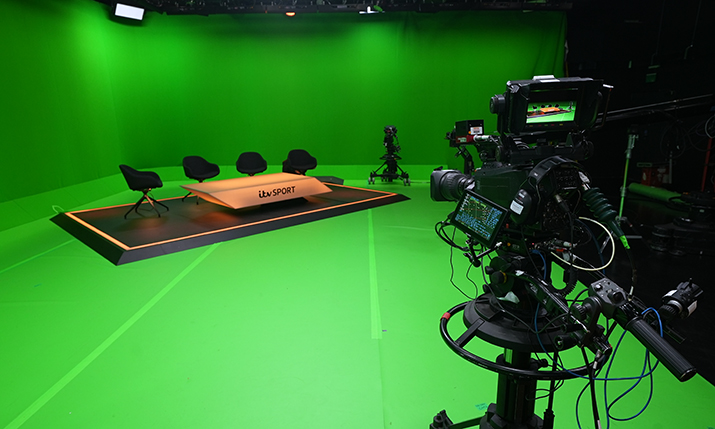The image captures a detailed view of a green screen studio designed for filming a sports show. The studio features green walls and floors, creating a seamless backdrop for digital edits. At the center of the setup is a slightly raised, black rectangular platform with red outlines. Atop this platform sits a white, three-dimensional parallelogram table branded with "ITV Sport" in black lettering. Surrounding the table are four black chairs, ready for guests or hosts.

On the right side of the image, a large television camera equipped with a digital screen shows the live view of what the camera is capturing. Another camera can be seen further back, positioned to the side of the platform, likely for additional angles. An overhead bright light is focused on the staging area, ensuring the set is well-lit for recording.

The left side of the image hints at more equipment or possibly an exit area, but the details are obscured by darkness. Overall, the image portrays a high-tech studio environment prepped for a professional sports broadcast, with all elements in place for a dynamic filming session.